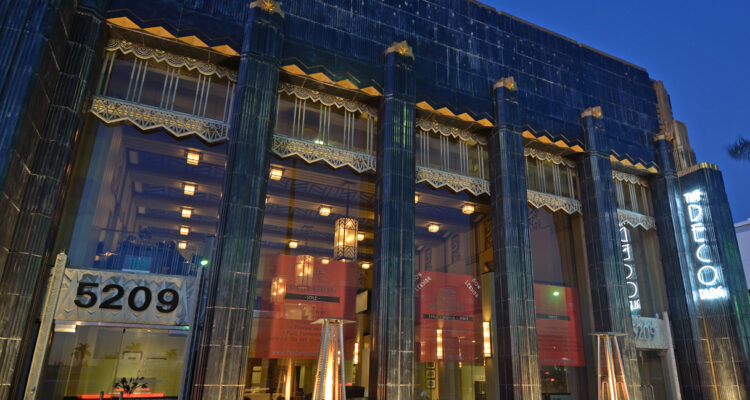This nighttime street view captures a striking building framed against a medium-dark blue sky, typical of city skylines at dusk. The structure, which spans almost the entire width of the image, is composed of a dark, grayish-black stone accented with streaks from mineral stains. The facade of the building is dominated by five large, vertically aligned windows flanked by four pillars. Each pillar is topped with intricate, gold-tinted filigree, and below the windows hang metallic, cage-like drapery elements tinged in orange-yellow. Prominently displayed on the left side of the building is a placard bearing the black-lettered address "5209." On the right side, a glowing neon sign reads "The Deco," casting a reflection on the adjacent window. Additionally, two brown stools are positioned in front of the second and fourth windows from the left. Overall, the detailed architectural elements and nuanced lighting create a captivating cityscape scene.